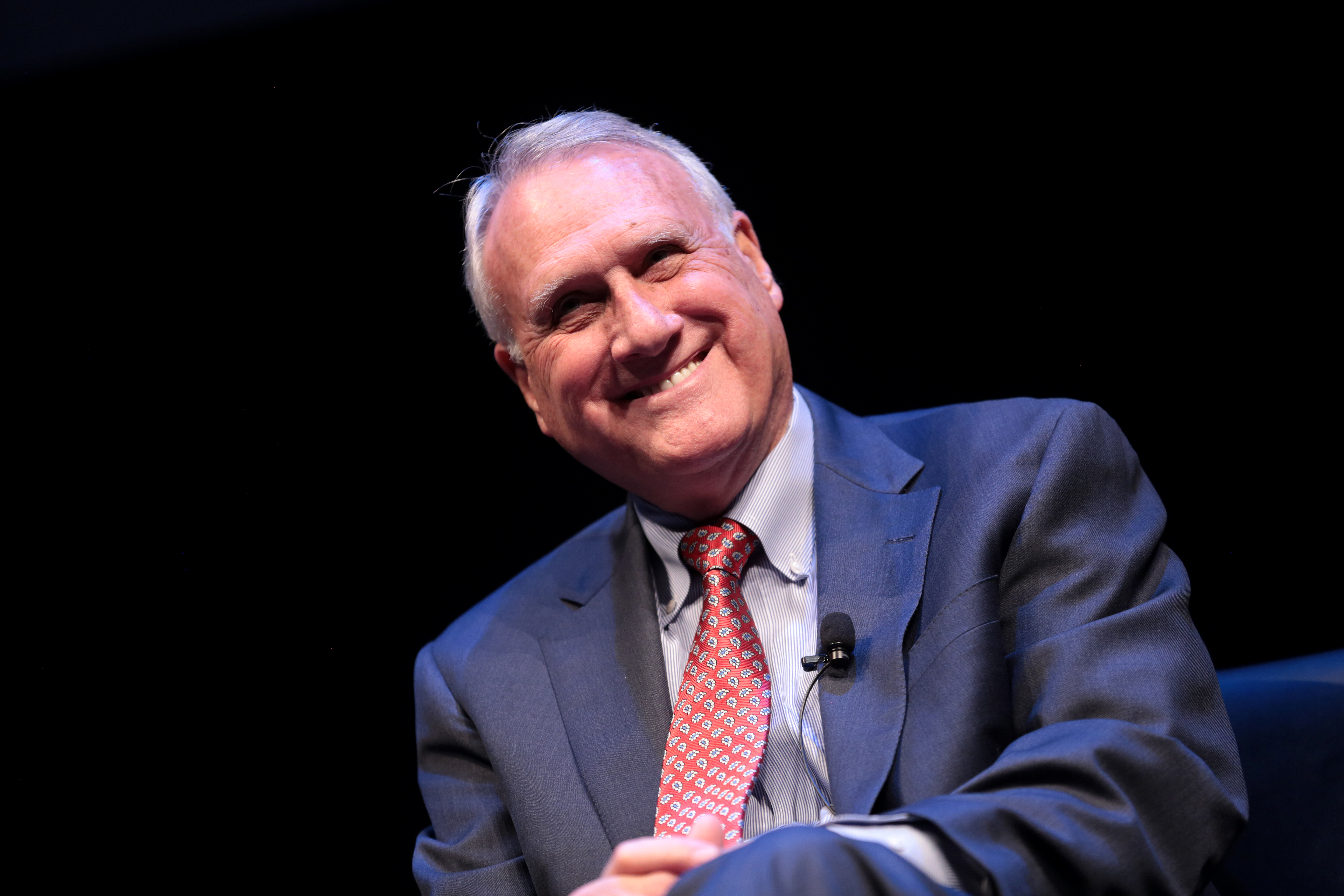In this detailed photograph, a man with white (or gray) hair is captured sitting against a solid black background. He is smiling warmly, partially revealing his teeth. He is dressed in a white button-down shirt paired with a blue coat and a red tie adorned with small blue and white spots. A black microphone is clipped to the left collar of his coat with a wire visible. The man's head and body are both tilted slightly to his right. His left leg is crossed over his right, but only the knee is visible as the rest of the leg is cut out of the frame. He is seated on a dark blue, cushioned sofa, a small part of which is visible behind him.